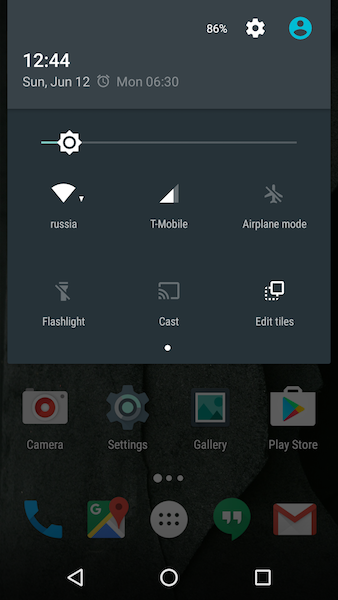This image showcases the quick settings panel of a Google phone, accessed by swiping down. Prominently displayed in the top left corner are large white numbers indicating the time as 12:44. Beneath this, the date, day, and time are listed alongside an alarm clock icon set for a future time. Below these details, a brightness slider is almost fully dimmed. Further down, the panel reveals a series of icons: the Wi-Fi icon labeled "Russia," indicating the connected network; a mobile signal icon showing connectivity to T-Mobile; and an airplane mode icon to the right, with "Airplane mode" written beneath it. The bottom row of icons includes a flashlight toggle, which is currently off, a cast icon, and an option to edit the tiles. In the background, the phone's home screen is partially visible, with various app icons scattered across it, including Camera, Settings, Gallery, Play Store, Google Maps, Hangouts, and Gmail.